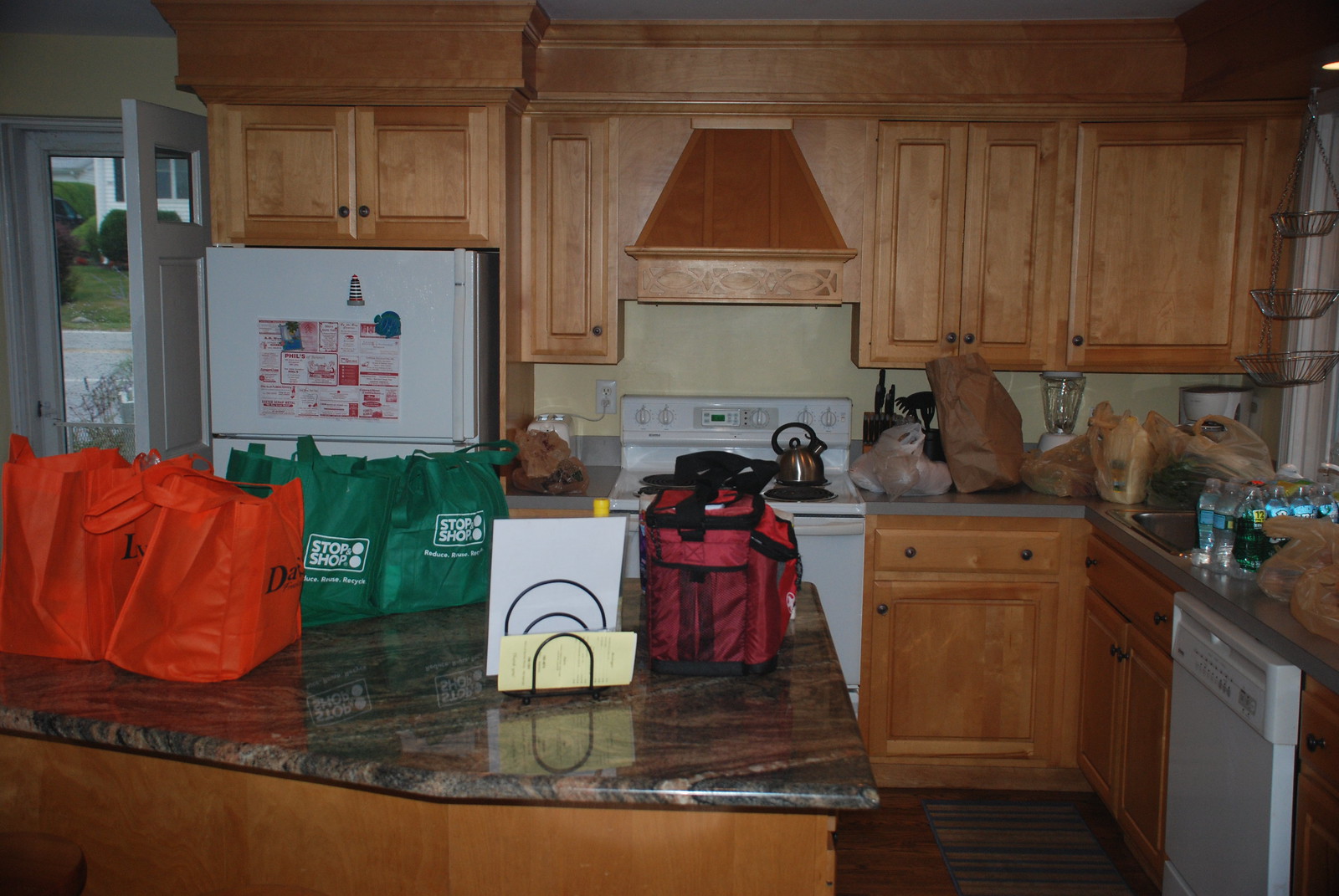A cozy indoor kitchen is captured in this photograph. In the upper left corner, the front door stands ajar, suggesting recent activity. Dominating the center of the room is a granite-topped kitchen island with a wooden cabinet base. On the island, there are two orange reusable cloth grocery bags with black lettering and two green bags displaying a white "Stop and Shop" logo. A white refrigerator, adorned with a blue magnet holding what appears to be a restaurant menu, occupies the left side of the photo. Above the fridge, brown wooden cabinets extend to the ceiling, finished with elegant crown molding. To the right, a white oven is flanked by gray Formica countertops, contrasting with the island’s granite surface. A white dishwasher is also visible. The kitchen floor features a wooden finish, partially covered by a rug, enhancing the room's warm and inviting ambiance.